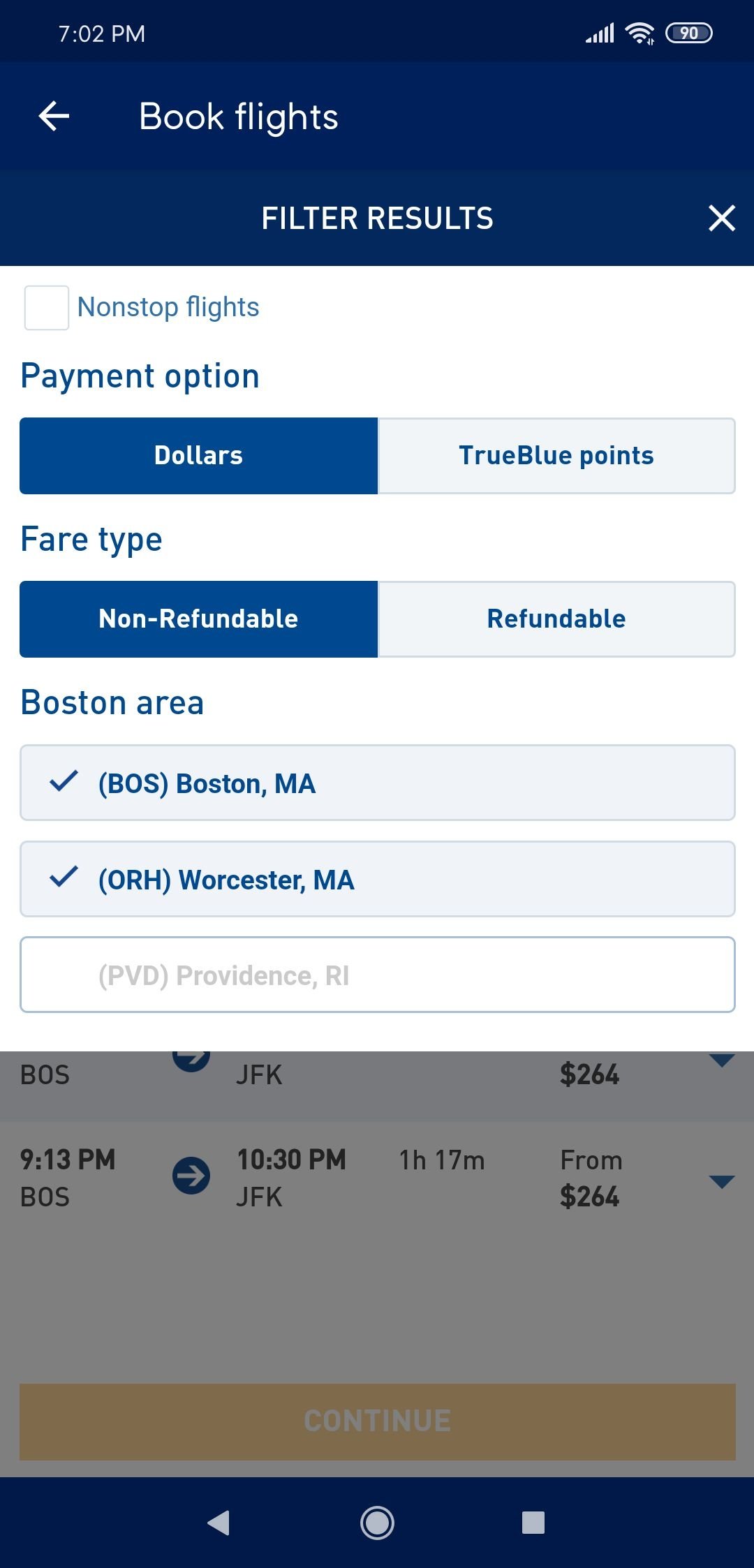This is a detailed screenshot captured from a cell phone displaying a flight booking website. At the very top is a black status bar where the time is indicated as 7:02 PM in the top left corner. On the top right, icons show the signal strength, Wi-Fi status, and battery percentage.

Beneath this, there is a dark navy toolbar featuring a white left-arrow icon for navigating back. In the center of this toolbar, the text "Book Flights" is also displayed in white. Directly below, there is another dark navy section centered with the text "Filter Results" in white, accompanied by a white "X" icon for closing the filter overlay.

The main section of the screenshot, with a white background, begins with the blue text "Non-Stop Flights." Following this is a bold header "Payment Option" with two selectable buttons: "Dollars" (displayed in white on a navy background) and "TrueBlue Points" (displayed in navy on a grey background).

Below this, another bold header "Fare Type" is shown. It is followed by two additional buttons: a navy button labeled "Non-Refundable" in white, and a grey button labeled "Refundable" in navy.

Beneath that section, the bold text "Boston Area" appears. There are two grey blocks with checkmarks; the first block indicates "BOS Boston, MA" and the second one indicates "ORH Worcester, MA."

A shaded background behind the pop-up suggests that another screen was already open, displaying some flight details. At the very bottom of this secondary screen, the navigation icons— a left-facing triangle, a circular icon in the center, and a square on the right—indicate that this screenshot was taken on an Android phone.